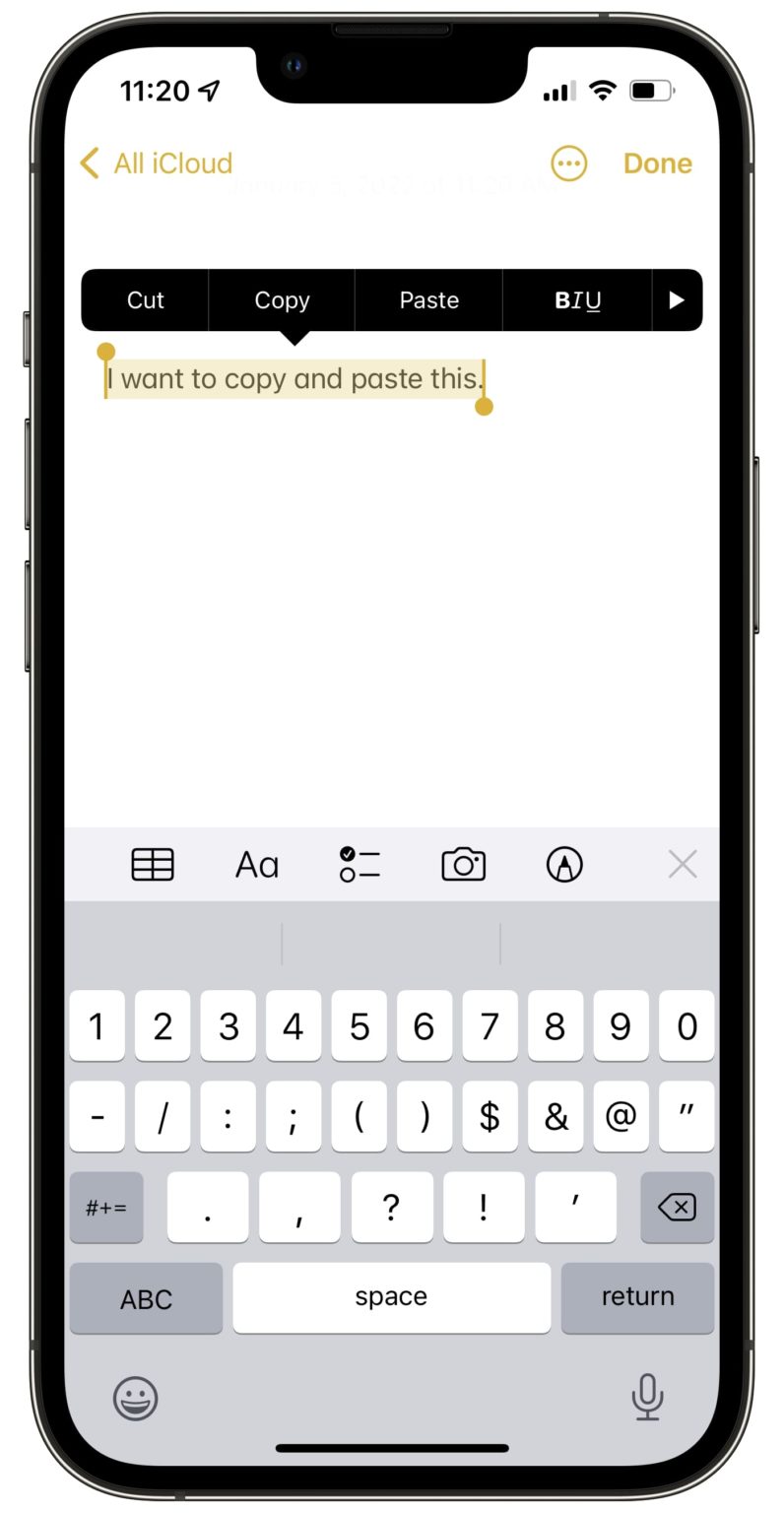This image features a smartphone with a generic black frame, characterized by its rectangular shape in portrait orientation and rounded edges. The phone has a trio of side buttons: a small top button and two longer buttons below, likely for volume control.

On the screen, the display boasts several details:

- At the top, in black font, the time is displayed as "11:20", complemented by a navigation arrow pointing to the top-right corner.
- To the right, status indicators include a three-out-of-four bar network connection strength, a fully lit Wi-Fi meter, and a battery icon indicating it is slightly over 50% charged.

Beneath these indicators is a gold-colored navigation bar. This includes a left-pointing arrow, followed by the text "All iCloud", a circle with three dots inside, and a "Done" button, all in the same gold hue.

Further down, there's a black pop-up text bubble with white font options such as "Cut", "Copy", "Paste", as well as formatting options: bold, italicize, underline, and a right arrow for more choices.

Highlighted in a pink-like border with additional gold accents, a line of black text reads: "I want to copy and paste this", indicating it is selected.

At the bottom, the on-screen keyboard is visible, displaying numerical keys.